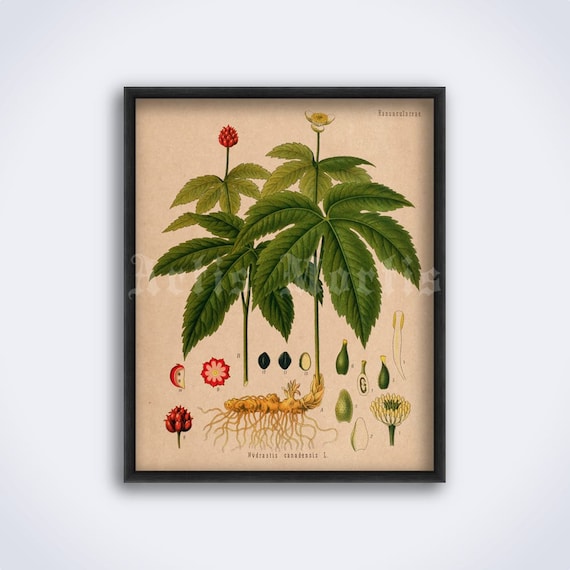This image is a photograph taken indoors of a framed vintage botanical illustration, reminiscent of those found in old botany or nature books from the 1800s or early 1900s. The photograph itself is square, about four inches in height and width, with a thin black frame, roughly an eighth of an inch thick. The illustration within the frame is on light tan background paper and depicts a detailed study of a plant, possibly a ginger plant, characterized by its extensive, yellowish root system. Emerging from the root are two tall, green stems crowned with large, fan-like, serrated leaves. The plant displays two distinct types of flowers: one stem supports a cluster of red bulbous flowers, almost berry-like, while the other features a white flower with a yellow center. Below the main illustration, there are detailed depictions of the individual parts of the plant, including cutaways of the red bulb and the white flower, as well as views of seeds and different floral structures. The composition is meticulously labeled, though the text is too small to read clearly in the photograph. The entire piece is mounted against a pale blueish-gray wall, suggesting a clean, indoor setting.